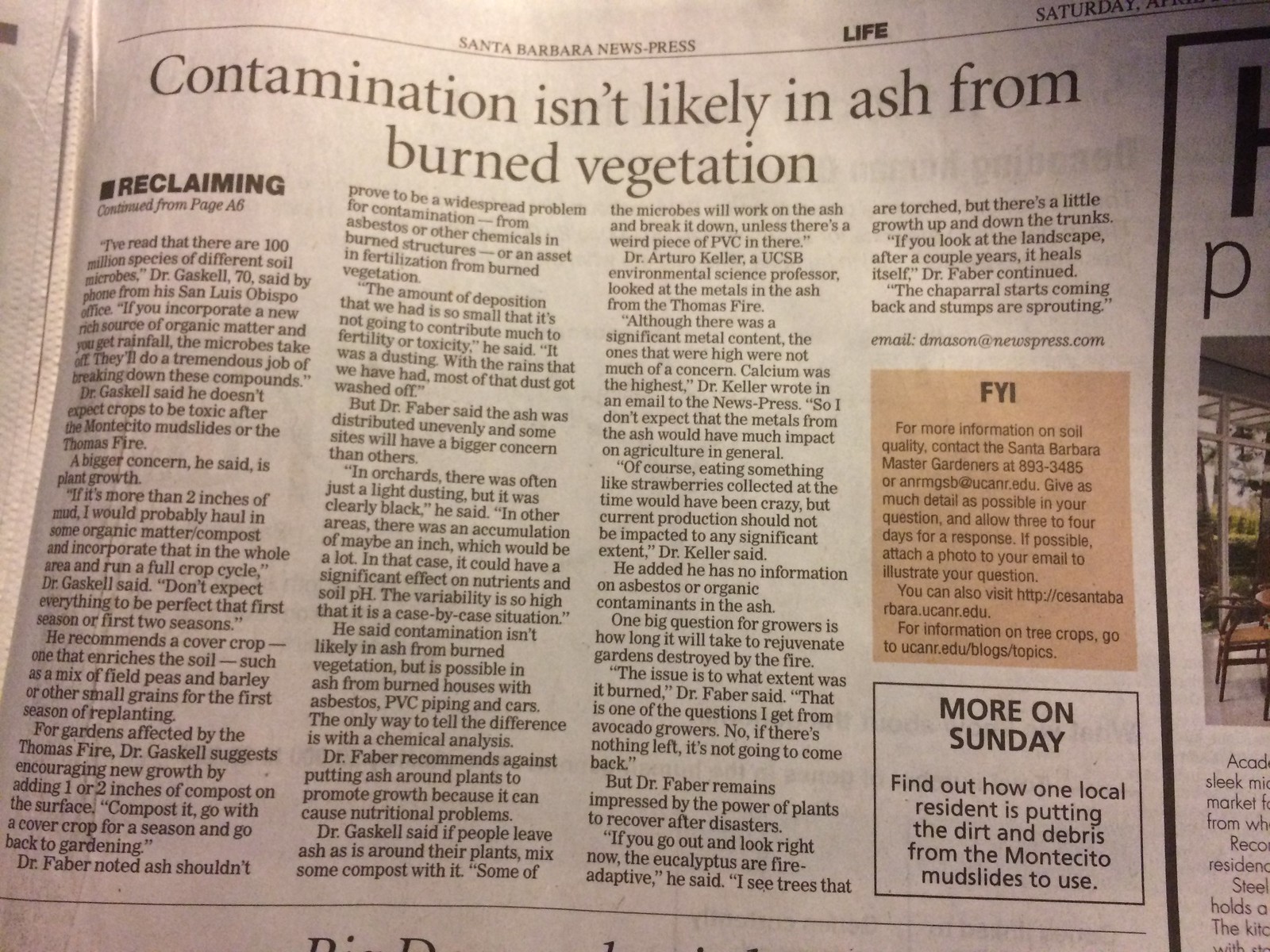The image depicts a wide rectangular photograph of a newspaper article from the "Santa Barbara News-Press," evident from the small black letters at the top, with a bold "Life" section designation next to it. The newspaper page has a light, almost white appearance with sections that show creases and corners indicating handling and age. The article spans four columns and is headlined in bold font: "Contamination Isn't Likely in Ash from Burned Vegetation." Beneath this headline, a portion of the article features a continuation from page A6, quoting Dr. Gaskell, a 70-year-old expert from San Luis Obispo, discussing the role of soil microbes in decomposing organic matter after rainfall.

Additionally, the right-hand side of the article hosts a tan-colored "FYI" box with another smaller black-bordered box below it. The latter box includes text reading, "More on Sunday," and hints at an upcoming story about local efforts in Montecito to repurpose dirt and debris from mudslides. Below the main title, the labeled continuation part "Reclaiming" indicates that the story had started on an earlier page.